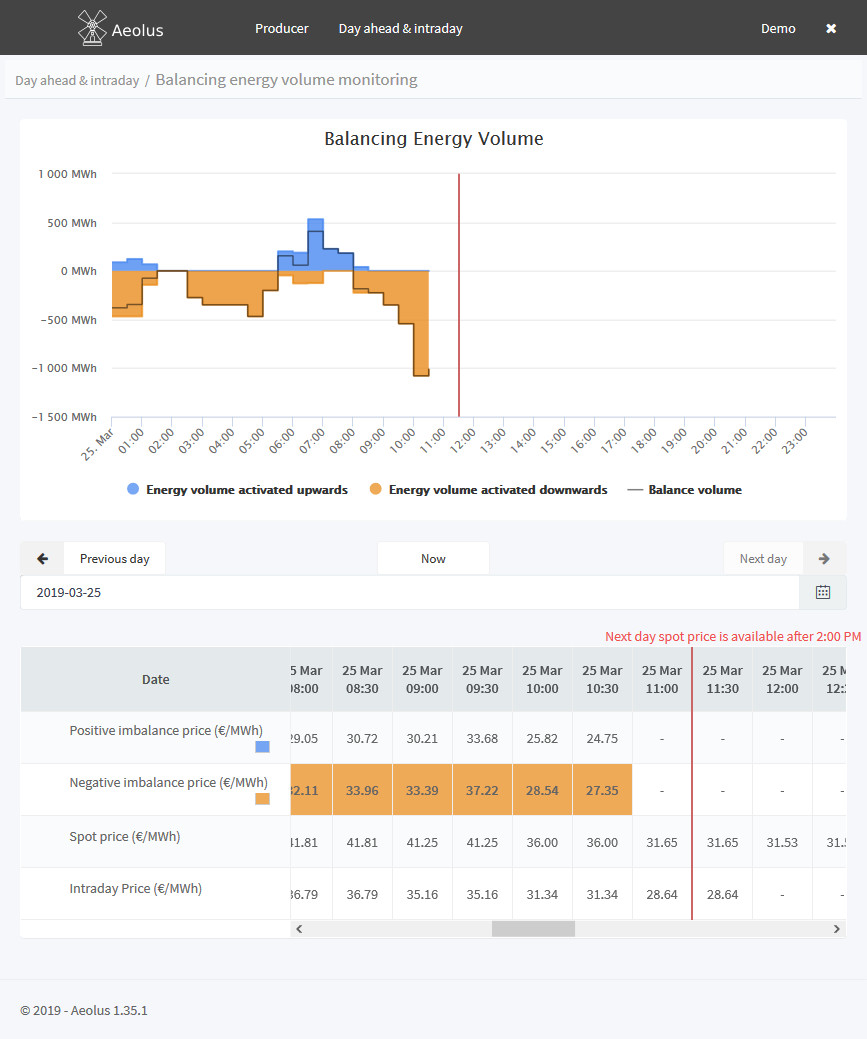This screenshot showcases a page featuring multiple data visualizations. At the top, a black menu bar spans the width of the page. On the left side of the menu bar, the title "AOLUS" is displayed alongside a windmill icon. Centrally located on the menu bar are two navigational links labeled "Producer" and "Day Ahead and Intraday." On the far right, there is a "Demo" link followed by a white 'X' icon.

Beneath the menu bar, two distinct charts are presented. The first chart, titled "Balancing Energy Volume," is a bar chart. It uses orange bars to indicate negative values and blue bars to highlight positive values. The X-axis is labeled from -1500 megawatt-hours on the left to +1000 megawatt-hours on both the bottom and the top of the chart. This chart likely visualizes the balancing of energy supply and demand, with the bars representing varying volumes of energy over a specific time period.